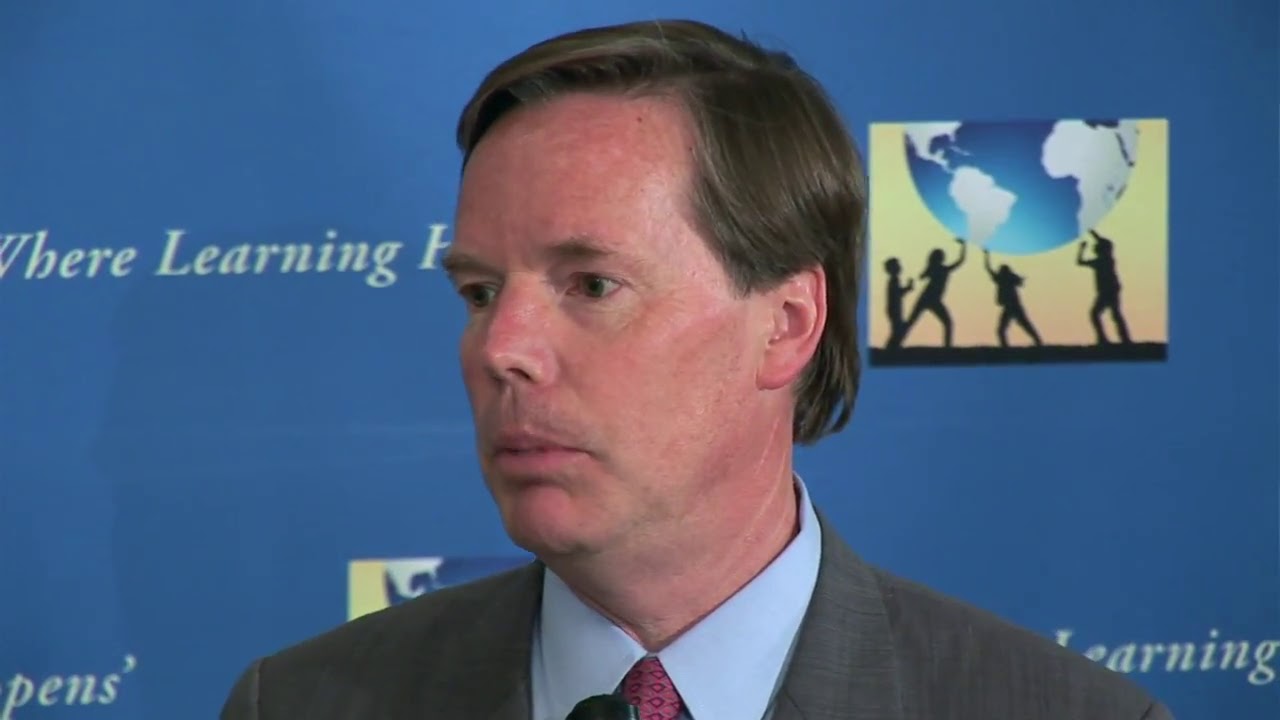In the center of the image is a man, presumably in his 40s, dressed in a sharp ensemble that includes a light blue shirt and a maroon tie, though some descriptions mention a pink tie. He is donning a gray suit coat. The image captures him from the upper chest upwards, emphasizing his short brown hair, which is combed to one side. His face appears slightly flushed and splotchy, and he is gazing slightly to his right without a distinct expression. The background is a blue wall, illuminated slightly, adding depth to the scene.

To the right of the man’s head is a partially visible poster depicting four figures holding up a representation of the Earth, which features blue oceans and white continents. This illustration is highlighted against a yellow background, providing contrast. To the left of his head, partially obscured by his position, are the words "we’re learning," suggesting the presence of more text that isn't entirely legible. Additionally, near his left shoulder is the end of a word, indicated by the letters P-E-N-S, and next to his right shoulder is the partial word "learning" with the "L" and "E" slightly cut off. This blend of visual and textual elements frames the man against an intricate and informative backdrop.